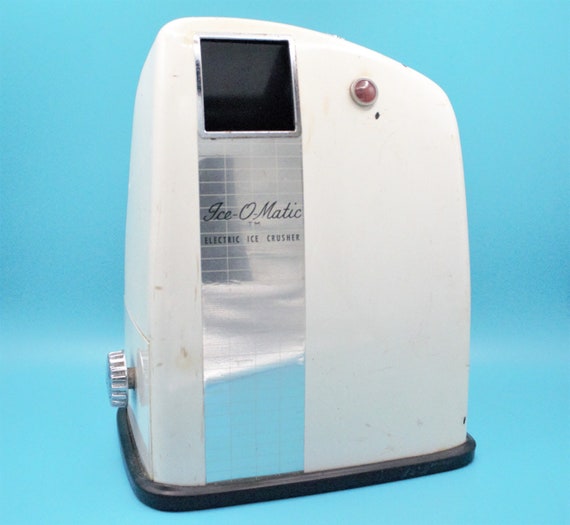The image showcases a vintage Ice-O-Matic electric ice crusher from the 70s or 80s, set against a uniform light blue background that appears to be both the surface and backdrop. The machine, predominantly white with a slightly irregular rectangular shape, features a black screen at the top left, encased in a shiny silver metallic frame. A label on the front left side, also in silver, clearly displays the brand "Ice-O-Matic" and the function "electric ice crusher" in black text. Below the screen, there's a small red light, currently off. The appliance's base is black, possibly plastic, encircling the entire bottom. The left-hand side of the machine has a silver, metallic dial. The overall lighting comes from the top, casting a slight shadow to the right. Slight hints suggest that ice might be inserted at the top, and there’s possibly a chute for dispensing crushed ice.